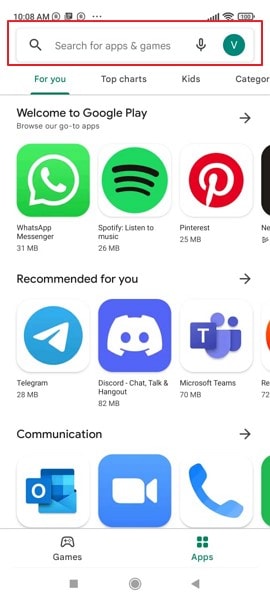The image is a screenshot captured from the display of a mobile phone, showcasing the Google Play Store's interface. At the very top of the screen, the time is prominently displayed as 10:08 a.m., accompanied by the battery icon indicating a full charge at 100%. Standard status icons such as the Wi-Fi signal and cellular network bars are also visible.

In the background, faint circular patterns add an aesthetic touch to the display. A red outline encircles the "Search for apps & games" section, giving it a distinctive rectangular shape. Within this outlined section, there is a small green circle featuring a 'V' symbol.

Beneath this search bar, the interface greets the user with the text "Welcome to Google Play" followed by options to "Browse" or "Go to apps." As you scroll down, several app listings are visible. "WhatsApp" and "WhatsApp Messenger" are listed first, with a size of 31 MB. Next, "Spotify" is available for download, with a file size of 26 MB. Following Spotify, "Pinterest" is listed, identifiable by the letter 'P' in a red circle, with a size of 25 MB. The subsequent app listing is partially visible and cut off.

Further down, the section titled "Recommended for you" appears, suggesting various apps under the category "Communication."